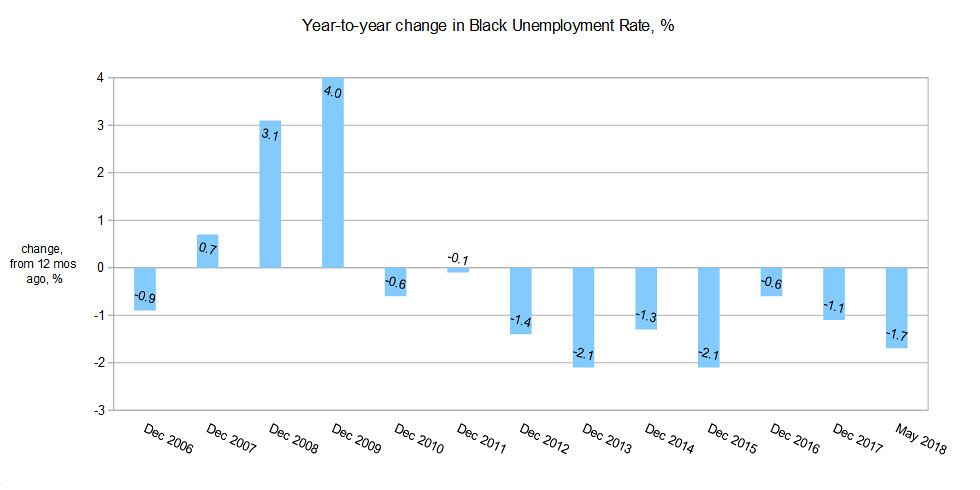The image features a bar chart on a white background, depicting the year-to-year percentage change in the black unemployment rate from December 2006 to May 2018. The text at the top of the chart reads in black font: "Year-to-year Change in Black Unemployment Rate, Change from 12 Months Ago, Percentage." The vertical axis on the left is labeled from 4 to -3, indicating the percentage change, while the horizontal axis at the bottom lists the years from December 2006 to May 2018. A horizontal line at the center indicates the zero percent change mark, with light blue bars extending either above or below this line to represent increases or decreases in the unemployment rate. The overall aesthetic appears professional, suitable for government or news-related contexts.